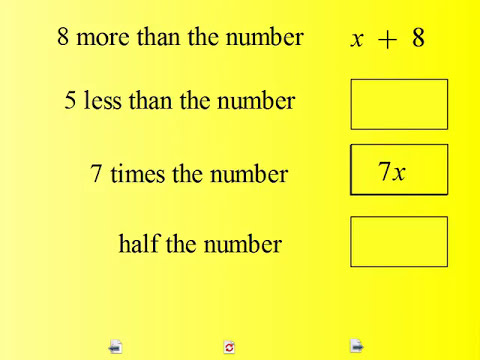The image appears to be a slide from a PowerPoint presentation or a projected overhead used for math teaching, specifically dealing with basic algebraic expressions. The background is a gradient, fading from yellow on the right side to almost white on the left. At the top, there are four lines of text in black font, each describing a mathematical expression with an accompanying box to the right:

1. "8 more than the number" with "x + 8" to its right.
2. "5 less than the number" with an empty rectangular box to its right.
3. "7 times the number" with "7x" in the box to its right.
4. "Half the number" with an empty rectangular box to its right.

At the bottom of the slide, there are three icons or buttons that resemble navigation controls: 
1. A sheet of paper with a blue arrow pointing left.
2. A refresh/reload symbol with curved arrows, one pointing right and the mirrored one beneath pointing left.
3. A sheet of paper with a blue arrow pointing right.

These icons suggest functionality for navigating through the presentation or slide set.